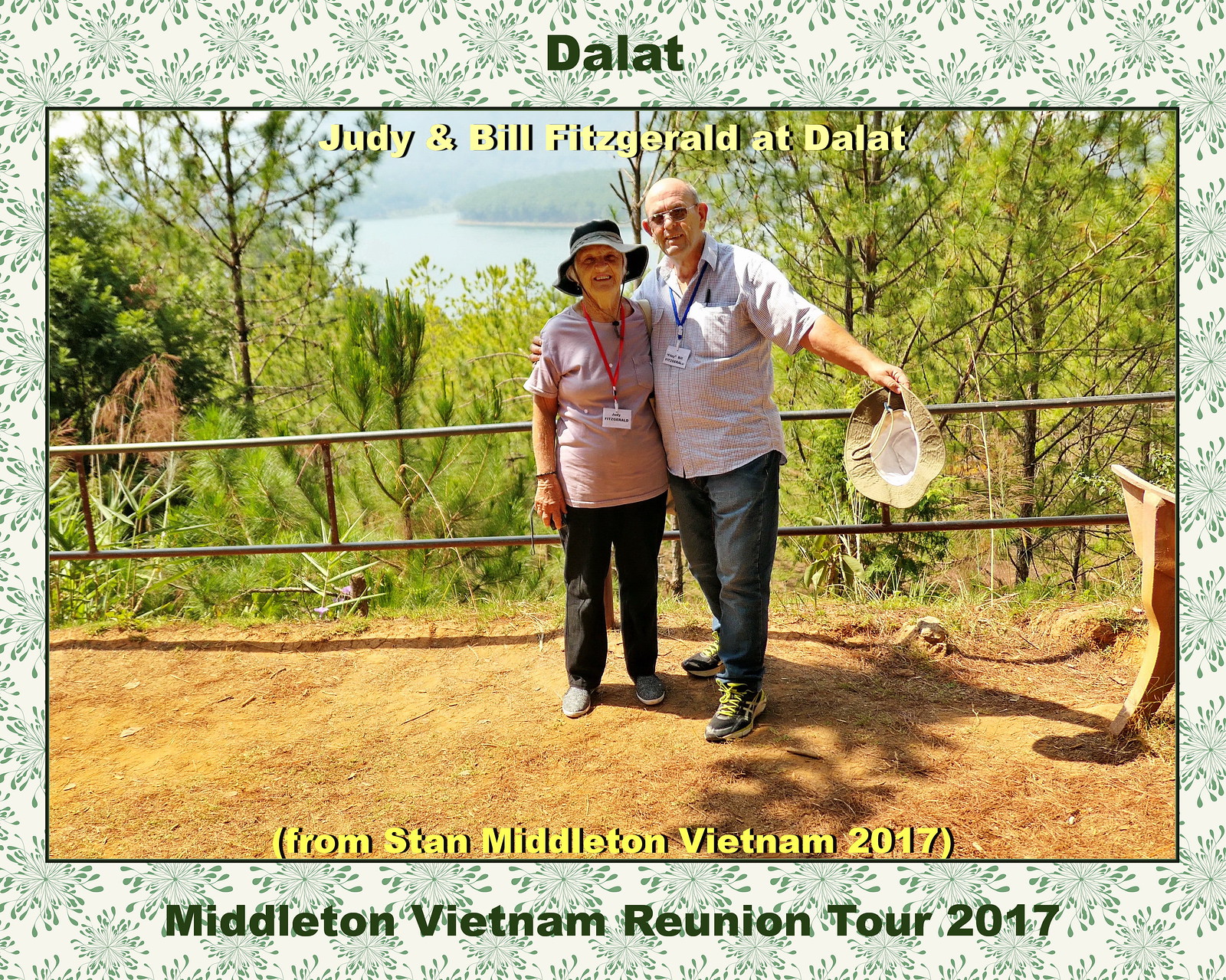The image depicts an older couple, Judy and Bill Fitzgerald, standing on a golden-colored dirt path, which appears to be a tourist destination in Dalat, Vietnam, as indicated by the green text "Dalat" at the top of the photo. The couple is dressed casually; Judy, positioned on the left, wears a light lavender short-sleeve t-shirt, a green hat, black pants, and black shoes with white bottoms. Around her neck hangs what appears to be a name tag on a red lanyard. Bill, on the right, sports sunglasses, a light-colored short-sleeve collared button-down shirt with blue striping, black pants, and black tennis shoes with yellow shoelaces and white bottoms. He extends his right arm outward, his hat facing towards the camera. The photo is bordered by a frame with a snowflake-like floral pattern. Behind them is a metal railing, a backdrop of evergreen trees, and a lake. Superimposed text within the photo caption at various points reads, "Judy and Bill Fitzgerald at Dalat," "From Stan Middleton, Vietnam, 2017," and at the bottom, "Middleton Vietnam Reunion Tour, 2017," emphasizing a reunion tour they were part of.